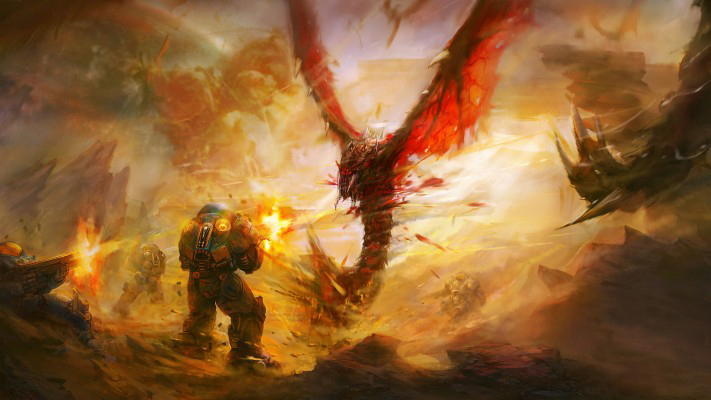This detailed illustration captures an intense battle scene, possibly from a game or a dystopian fantasy realm. In the foreground, we see the back of a heavily armored soldier, donned in a futuristic tech suit with tones of red, brown, and yellow. He wears a silver helmet and is firing a powerful gun, evidenced by the blazing yellow flame shooting out. His target is a massive, grotesque creature reminiscent of a dragon or flying demon, characterized by its enormous red wings streaked with veins of brown or black, a shrimp-like body and tail, a silver snout, and sharp claws and teeth. The monster’s body is a mix of reds, blacks, and yellows, with blood spurting from it as it's hit.

Behind the primary soldier, there's another warrior partially visible, their gun also emitting a bright flame with yellow and orange hues. The chaotic background is lit with murky tones of yellow, orange, and purple, suggesting that the environment is ablaze. To the right, another dark, dragon-like creature with a glowing yellow eye and pointed features looms menacingly.

The scene also depicts a hilly, sandy terrain beneath the combatants, adding to the apocalyptic atmosphere. Further back, other robotic soldiers and monstrous figures, possibly large rhino-like beasts, can be seen, contributing to the sense of a widespread, ongoing battle. This vivid portrayal combines elements of futuristic warfare with a nightmarish fantasy, emphasizing the relentless struggle between the armored soldiers and their monstrous adversaries.